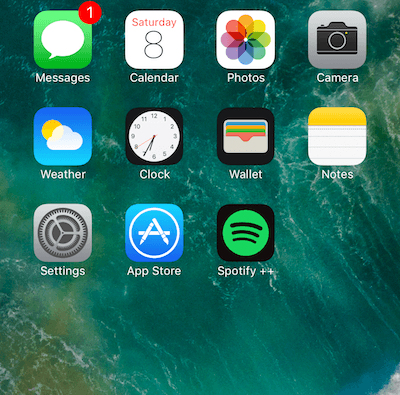The image captures the home screen of a mobile device, set against a serene background featuring sea green water with gentle, white foamy wave patterns. The app icons are neatly organized in three rows; the top two rows each contain four icons, while the bottom row houses three icons.

In the first row, from left to right:
1. A messaging app icon depicts a white speech bubble within a green square with rounded corners. A small red circle with the number '1' signifies one unread message.
2. The calendar app icon displays the word "Saturday" and the number "8."
3. The photos app icon, likely representing a photo gallery.
4. The camera app icon, indicating quick access to the camera function.

The overall composition of the home screen is visually appealing and meticulously organized, providing a user-friendly interface.